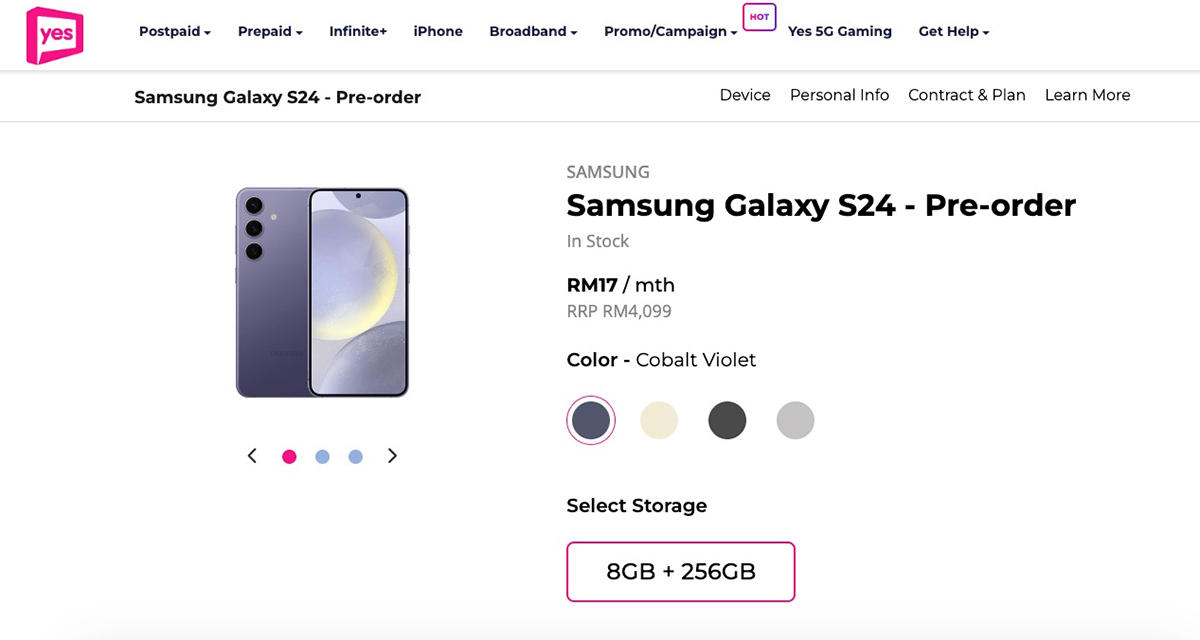The image depicts a webpage with a predominantly white background. In the top left corner is a square pink logo on a white background featuring the word "Yes" in pink. The header of the page contains multiple navigation tabs with drop-down menus: "Post-Paid," "Prepaid," "Infinite Plus," "iPhone," "Broadband," and "Promo/Campaign." Next to these, there's a prominent "HOT" indicator in a pink and purple square. Additional tabs include "Yes," "5G Gaming," and "Get Help."

In the body of the webpage, there is a headline in black text announcing the "Samsung Galaxy S24 Pre-Order." Beneath this headline are more tabs labeled "Device," "Personal Info," "Contract and Plan," and "Learn More."

The central feature of the page is a detailed image of an Android device showcasing both its front and back. The device is rectangular with three rear cameras aligned in a row next to a white flash. The front display screen exhibits various circular icons. The device is available in at least three colors: pink, blue, and light blue, suggesting additional color options may be available.